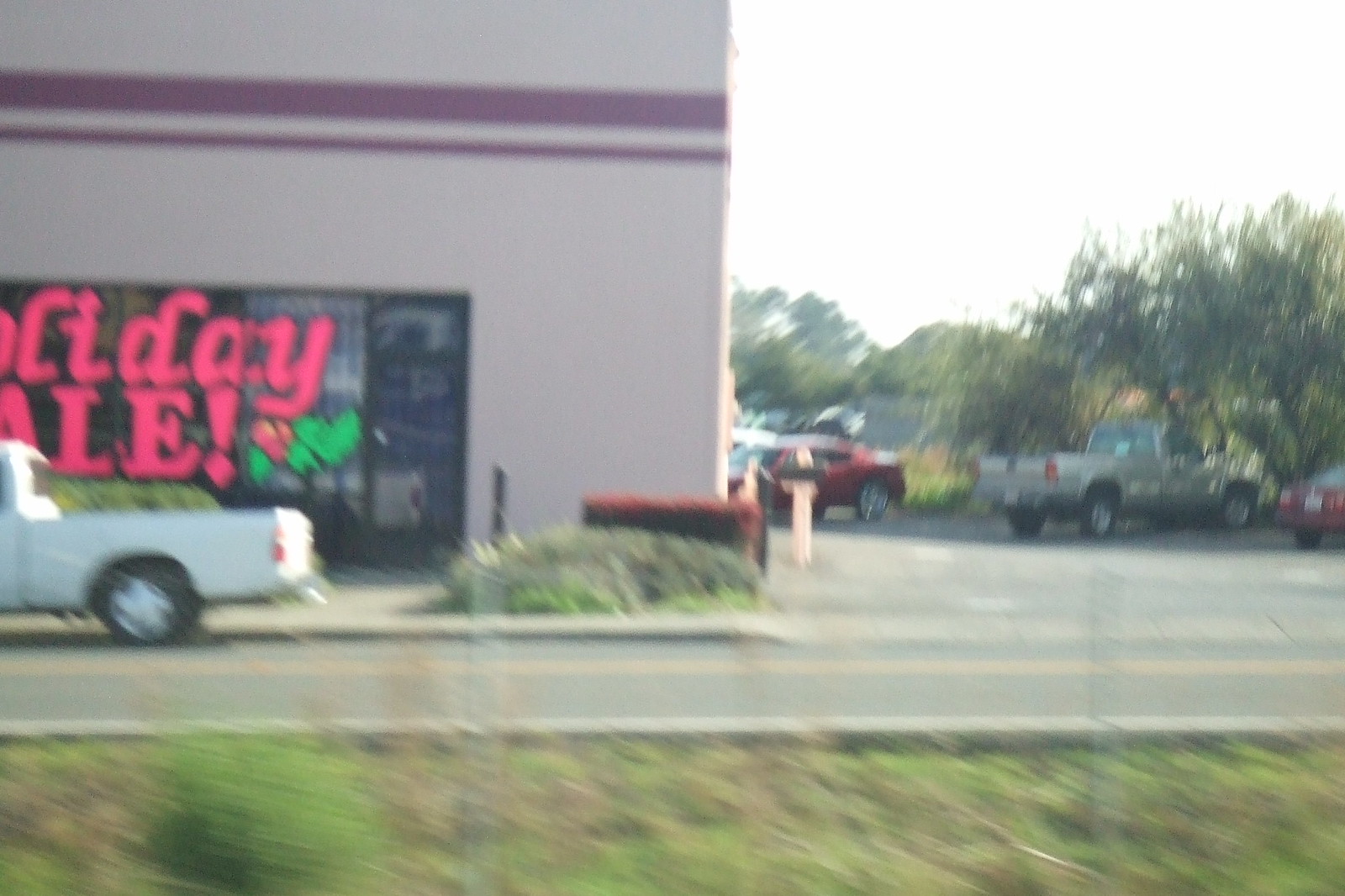This image captures a somewhat blurry photograph of a two-lane roadway bordered by a semi-grassy, semi-dirt area with a green and brown patch of grass, a small green bush, and a curb. The road features a double yellow line down the center. To the left of the image, a white pickup truck is either driving or parked towards the left side of the road.

Occupying the back left-hand side of the photograph is a beige (ivory-colored) building with red (brown) trim and bright pink lettering that reads "Holiday Sale" on the storefront windows. The building also displays green leaves and red berries as part of the decoration. In front of the store, there is a small bush area adding to the festive display.

To the right of the building, the image shows a parking lot with two cars and a truck parked, with trees lining the back of the parking area. The sky above is clear, giving a complete view of the business and its surroundings.